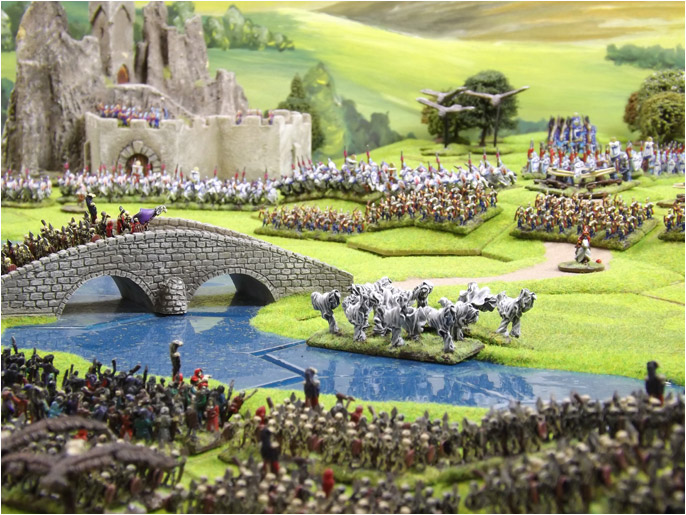This detailed painting depicts a whimsical, almost cartoonish medieval battlefield scene, vividly brought to life through imaginative toy-like figures. The composition features numerous troops spread out over a vivid, fake green grass landscape, assembled along both sides of a sparkling blue river. A stone-like bridge stretches across the river, with soldiers parading halfway across it while others prepare strategically on the bank. In stark contrast to the playful demeanor of the figures, a grand, though somewhat worn-looking stone castle stands prominently in the background, surrounded by rolling hills and stylized, painted trees. Additionally, a quaint pavilion, possibly hosting the commanders, is subtly tucked in the background. The troops are varied, comprising ground soldiers, and cavalry contingents with toy paladins mounted on horses, complete with spears and armor. Larger white animal statues, perhaps part of the creative ensemble, stand poised near the river, ready to metaphorically dive into the action. The sky is rendered in broad, expressive brushstrokes, contributing to the distinct artistic quality of the scene. Despite the playful, toy-like representation, the painting captures the essence of an impending medieval battle with rows of disciplined troops lined up meticulously, ready for confrontation.